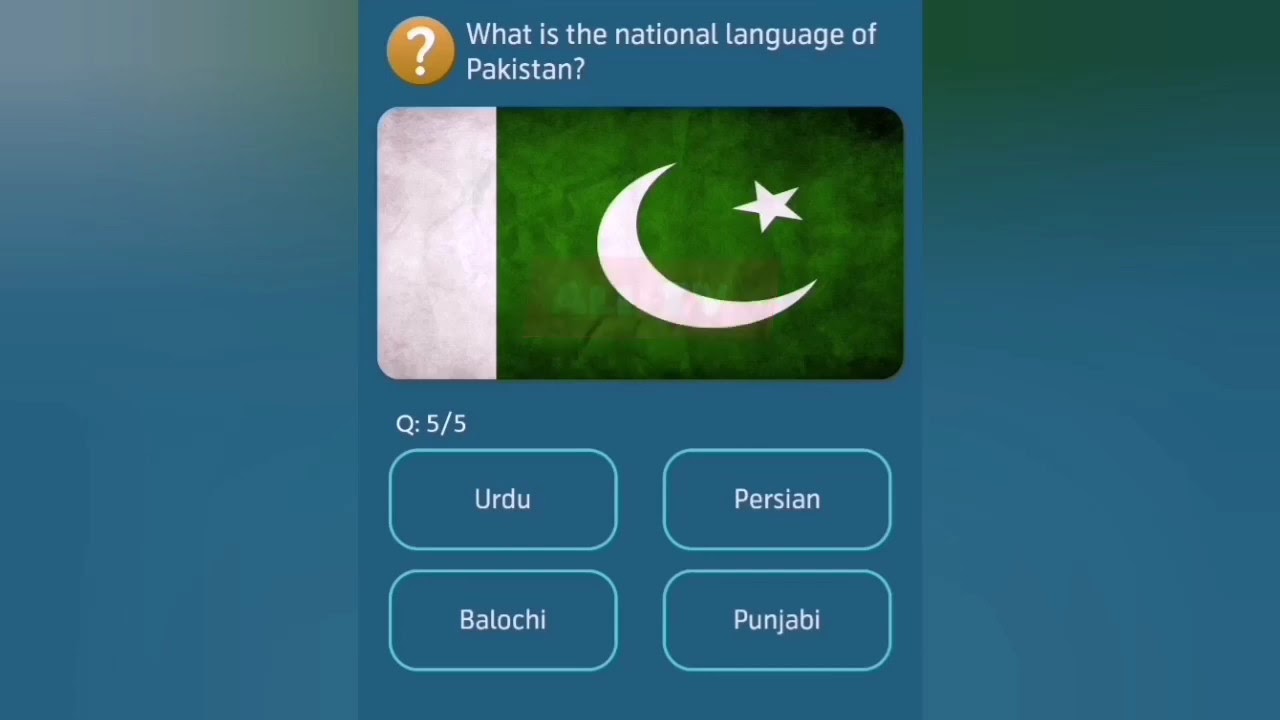The image is a screenshot of a quiz application, set against a light blue background. It prominently features a vertical rectangular area in the center, also with a blue background, though slightly different in shade. At the top of this central area, there is a white question mark enclosed in a circle followed by the question in white text: "What is the national language of Pakistan?" Directly below the question is an image of the Pakistani flag, which has a white strip on the left side taking up about 20% of the flag's width and a green area on the right. The green section features a white crescent moon with its ends pointing to the top left and bottom right, accompanied by a white star to the right and slightly above the crescent. Directly below the flag, there is an indicator showing "Q: 5/5," suggesting it is the fifth question out of five. Beneath this, there are four answer choices arranged in a two-by-two grid, each within a rectangular box with rounded edges and a light blue outline. The choices, written in white text, are: URDU, BALOCHI, PERSIAN, and PUNJABI.